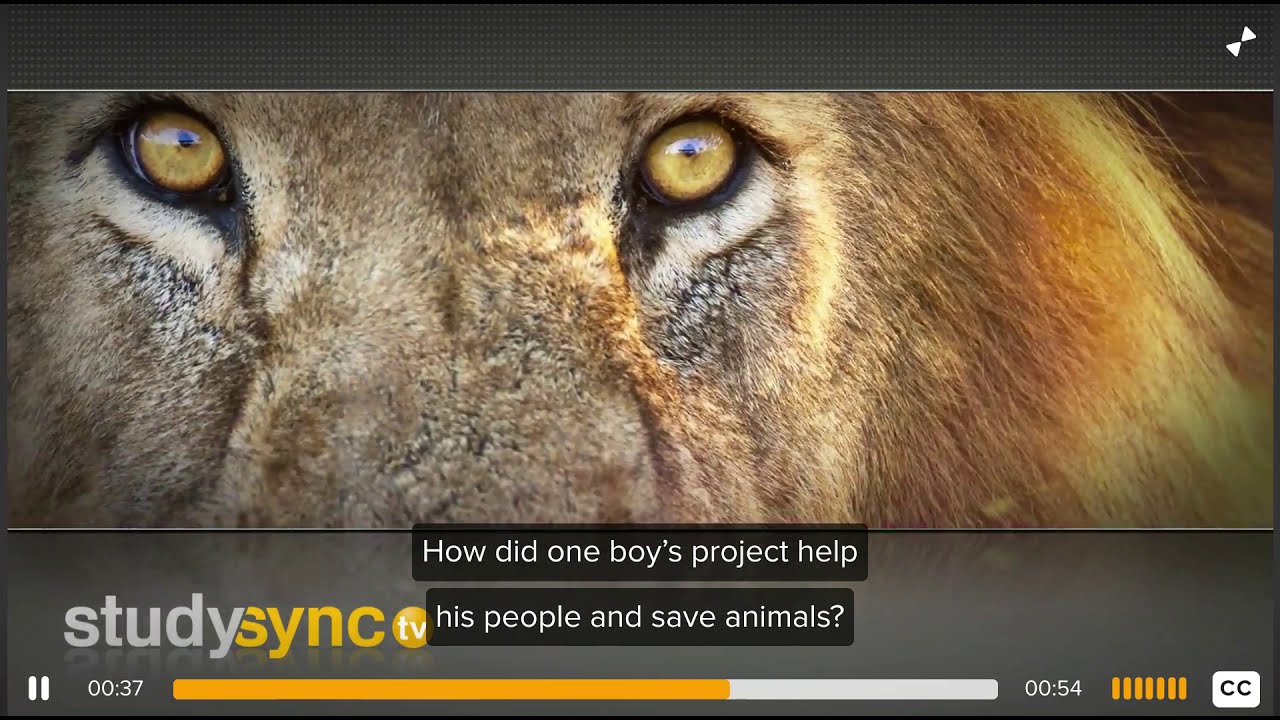This horizontally aligned rectangular image is a close-up of a lion's eyes, framed by a subtle patterned gray border that is thicker at the bottom than at the top. The image focuses on the lion's intense golden eyes, capturing the middle portion of its face and a bit of its mane on the right side, which is a mix of brown and gold with a hint of white underneath the eyes. At the bottom center, the text reads: "How did one boy's project help his people and save animals?" in white, centered over two lines. This appears to be a snapshot from a video, denoted by the video controls visible within the image. In the lower left corner, there are the two vertical bars of the pause button, next to the timestamp “00:37” out of “00:54.” A progress bar, primarily yellow with the remaining part white, runs below these timestamps. The lower right corner displays a "CC" symbol against a white square background, indicating closed captions. The implication is that this image is part of a commercial or educational video, possibly from "Study Sync TV," aiming to draw attention to the impactful project of a boy in aiding his community and protecting wildlife.